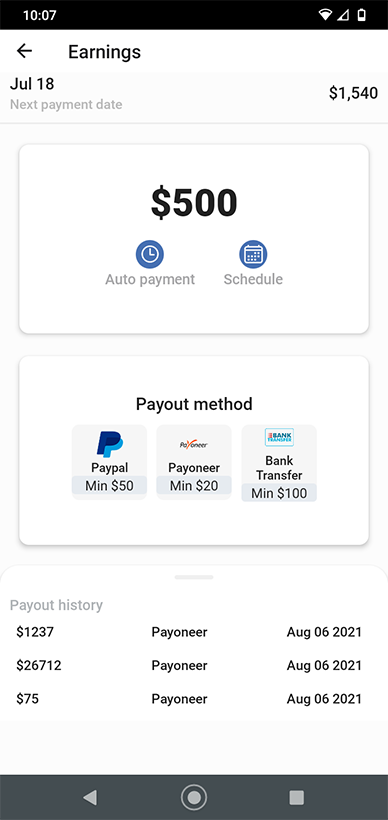The screenshot seems to be from a tablet or smartphone. At the top, the time reads "10:07" in military time format. The WiFi symbol is nearly full with about a third missing, the cell phone signal indicator shows about two-thirds missing, and the battery icon is approximately two-thirds depleted.

Below this status bar, set in a grayish-white background, there's a black arrow pointing to the left, followed by the bold black word "Earnings." Directly underneath, it displays "JUL 18," likely referring to July 18th, with an amount of $1540 shown on the right-hand side. Beneath this, in gray text, it mentions "Next Payment Date."

A dark gray line separates this section from the next. There is a large white rectangle in the center, containing bold black text displaying $500. Flanking this area, there are two circles: the left one features a clock face icon with the label "Auto Payment," and the right one shows a calendar icon with the label "Schedule." Both buttons are dark blue with white icons and text.

Further down is another white rectangle that reads "Payment Method" in bold black text. Below this are three payment method options:
- PayPal, with the PayPal logo and minimum amount of $50.
- Payoneer, represented by a logo that reads "PAY" with a cascading "Y" in orange, and a minimum amount of $20.
- Bank Transfer, identified by a cyan blue and dark blue icon, logo appearing red, and a minimum amount of $100.

At the bottom is the "Payout History" section, starting on the left and listing amounts in chronological order:
- $1,237
- $2,626,712
- $75 Payoneer, dated August 6th, 2021

Finally, the screen's bezel at the bottom displays three navigational elements: a white arrow pointing left, a circle with a semicircle outside of it in the center, and a square on the right-hand side.